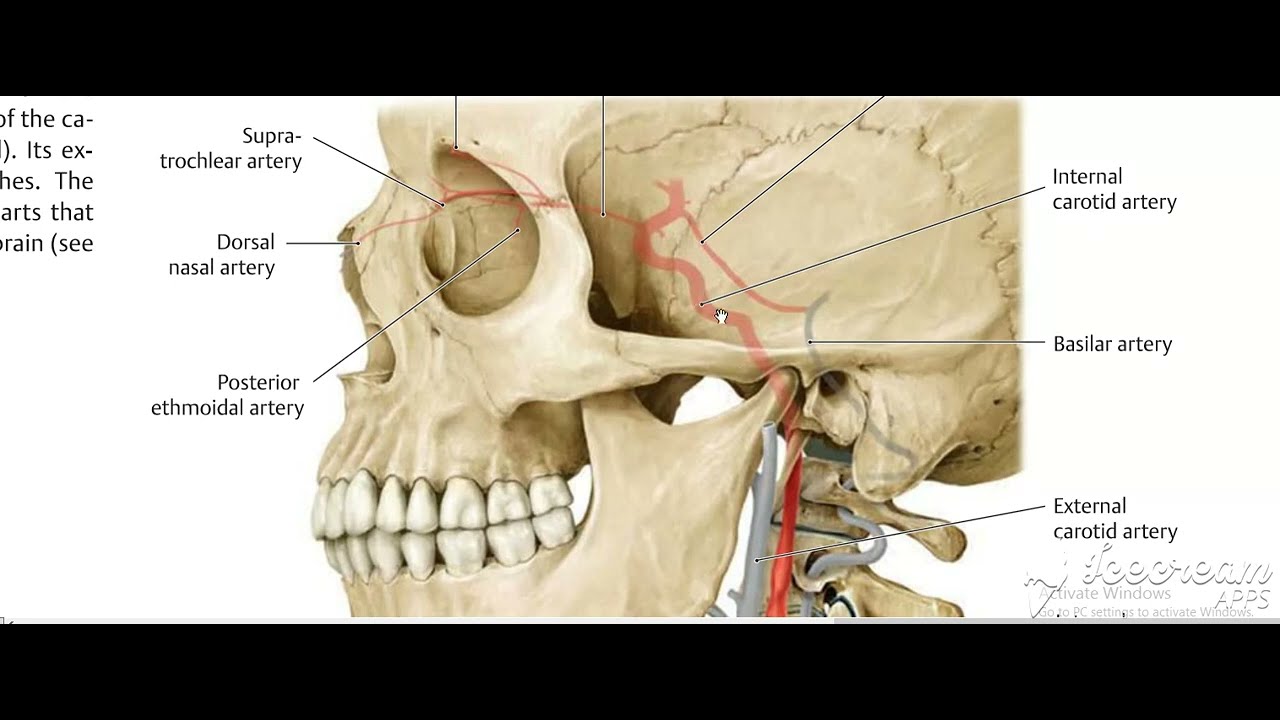The image is a full-color horizontal photograph of a human skull in profile, facing left. It features a thick black border at the top and bottom, but not on the sides, with a simple white background. In the lower right-hand corner, there is hard-to-read text mentioning something about "tea cream apps activate windows." The skull image extends from the jaw up to around the eyebrow level, revealing one eye socket, but does not show the very top of the skull. Various arteries within the skull are labeled with black lines pointing to their respective locations. These labels include the supratrochlear artery, dorsal nasal artery, posterior ethmoidal artery, internal carotid artery, basilar artery, and external carotid artery. The skull's teeth are prominently displayed, and overall, the image provides a detailed anatomical view of the vascular structure within the human skull.